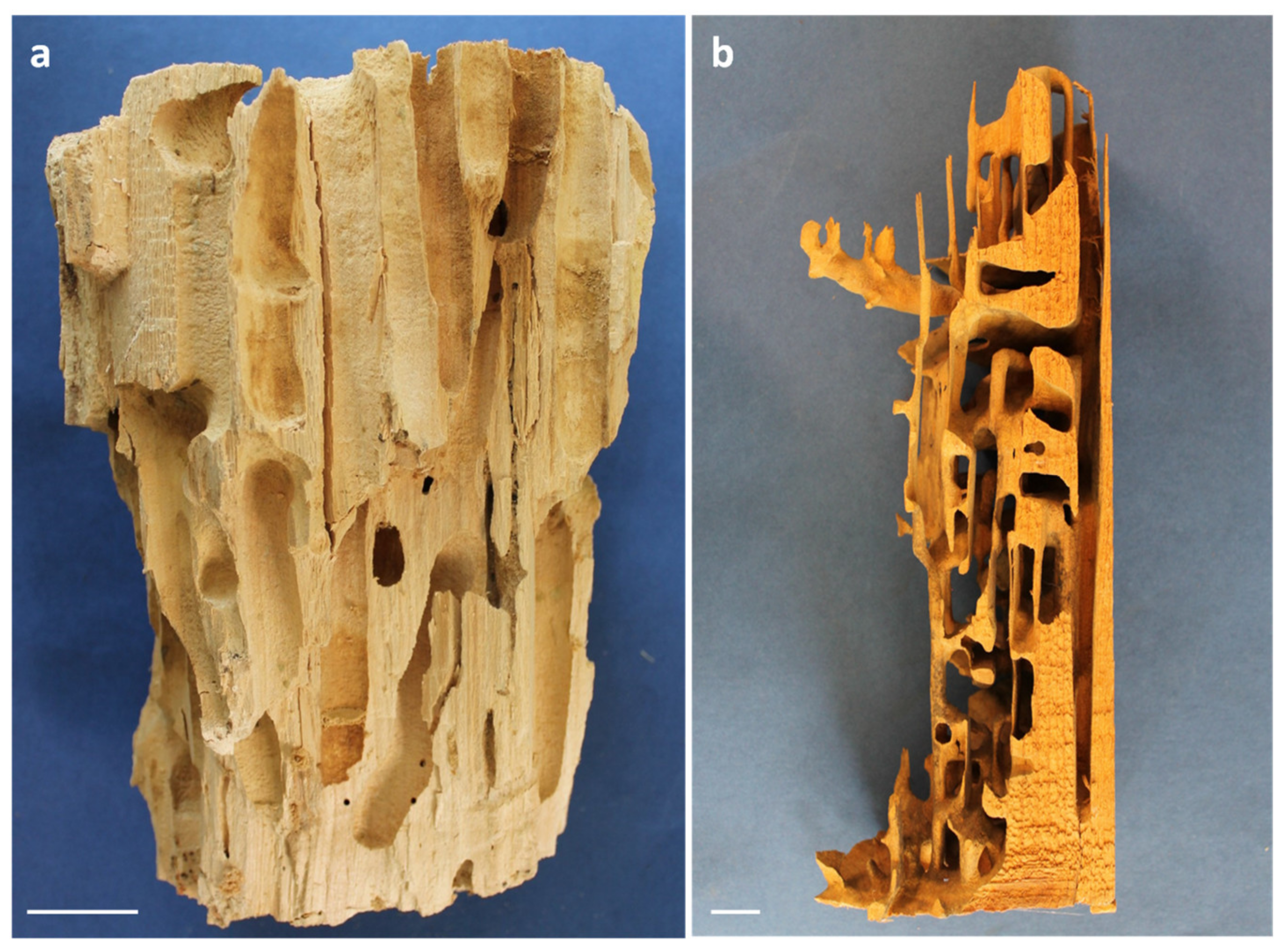The image is a split photograph resembling a museum exhibit, showcasing two distinct wooden sculptures against contrasting backgrounds. The left half, labeled "A" in white in the upper-right corner, features a textured, light-colored wooden piece with numerous holes and indentations reminiscent of a natural log. The background is a rich blue, and a small horizontal line underscores the label. The right half, labeled "B" in a similar white font, presents a more intricately carved, reddish-orange wooden sculpture, suggesting deliberate artistry and creativity. This piece appears meticulously whittled into a pattern or track, evoking a sense of playful functionality, as though designed for marbles to traverse through its ingeniously placed checkpoints and holes. The backdrop here is a striking gray, further highlighting the contrast between the two wooden objects.